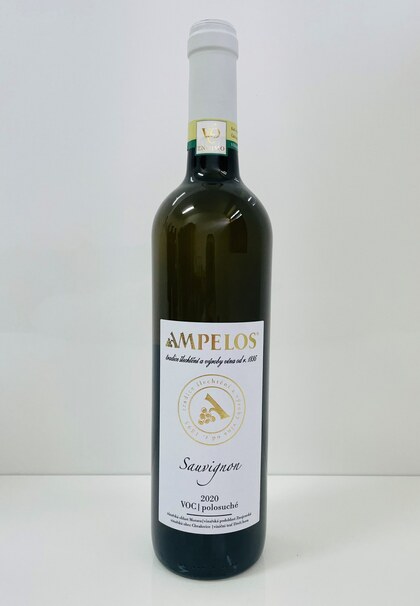The image portrays a professionally photographed bottle of wine suitable for a website display or sales picture. The backdrop is minimalist with a pristine white wall and a matching white table, emphasizing the bottle of wine as the central object. The bottle itself is a very dark green or nearly black glass, prominently situated in the middle of the frame within a vertical rectangular composition, approximately twice as tall as it is wide.

Adorning the bottle is a white foil wrapping at the top, with a distinctive yellow and green striped band circling the lower part of the neck. The main label is a large white and gold rectangular sticker that stands out starkly against the dark glass. At the top of this label, "Ampelos" is prominently inscribed in elegant gold lettering. Beneath this, "Sauvignon" is beautifully etched in black script, followed by "2020" in the same black font. The label also features sophisticated gold embellishments, including a circular drawing of a grapevine.

The sealed bottle, containing wine up to the neck as suggested, is impeccably centered against the monochrome background, making for a clean, sharp, and highly detailed image that highlights the luxurious appeal of the wine. The colors in the image include variations of white, black, green, yellow, and gold, contributing to a sense of elegance and high quality. 

Overall, the detailed description and the positioning of the elements make it ideal for a wine website, giving potential buyers a clear and enticing view of the product.